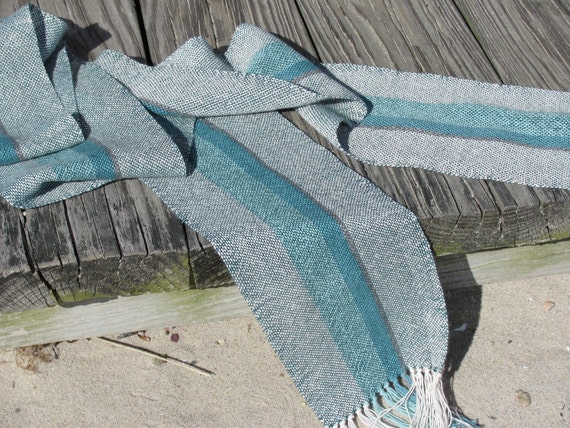The image features a long, wide scarf artfully spread out over a weathered, gray wood surface, likely a deck or table, with fine, light-colored sand visible underneath, hinting at an outdoor setting. The scarf showcases a striking combination of colors including hues of turquoise blue, lighter green-blue, bluish gray, dark gray, and gray, arranged in a striped or plaid pattern. The edges of the wood paneling are accentuated by light mossy green hues, adding a touch of natural contrast. The scarf, soft in appearance, is adorned with tassels that mirror its color palette—white, blue, and teal—offering a cohesive and appealing visual. The wood surface has a thick appearance with visible signs of age and wear, contributing to the rustic charm of the setting, further enhanced by sunlight gently illuminating the scene.